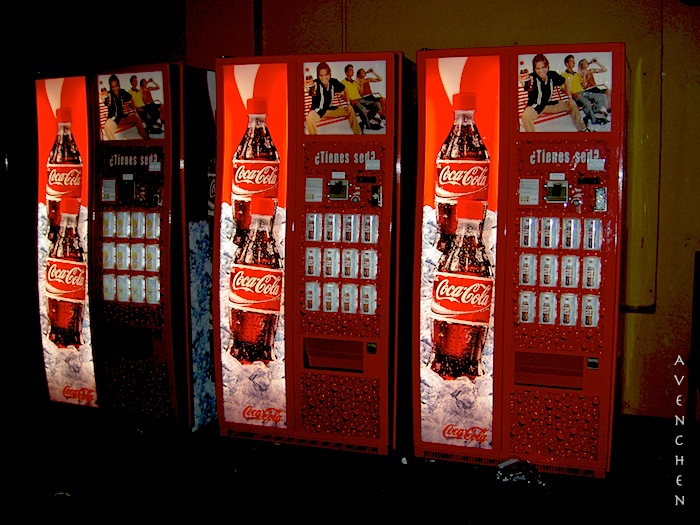The image showcases three identical Coca-Cola vending machines lined up against a yellow speckled wall with red accents. Each machine features a prominent left panel displaying two stacked plastic Coca-Cola bottles, set in ice with their iconic red labels. On the right panel, above the selection buttons, there's an image of three people—a female and two males—sitting on a park bench, drinking Coca-Cola. While all the machines share this visual consistency, the one on the far left uniquely offers various yellow-colored drink options, though the specifics are hard to discern. Notably, the vending machines primarily use red in their color scheme, contrasting with the dark, dimly lit floor.